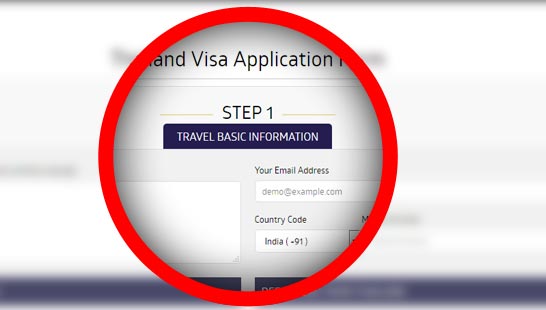This is an instructional image, possibly from a step-by-step or how-to guide. A large red circle in the middle of the image focuses on specific text, highlighting the relevant content while the rest of the image is blurred. The background of the entire image features a white and gray color scheme, with a few grayish boxes scattered around.

Inside the red circle, the highlighted text includes the following:

1. **Black Text: "Step One"** - This is prominently displayed and flanked by two gray lines on either side.
2. **Blue Box: "Travel Basic Information"** - Positioned beneath the "Step One" title, the blue box slightly extends beyond the text on both the left and right sides, and it is centered on the page.

At the top of the red circle, you can see portions of additional text, including fragments such as "A and D," "visa," and "application." However, parts of the text remain unclear.

Below "Step One: Travel Basic Information":

- A text box is located on the left side, though its header information is blurry.
- On the right side, there is a text box labeled for an email address, complete with a placeholder example email.
- Beneath these, another text box appears to hold a phone number, featuring fields for "country code" and a drop-down menu set to India, displaying "+91" (India's international dialing prefix).

The text boxes within this section are white, contrasted against their gray background, and their headers are in black font.

![Instructional Image Highlighting Step One: Travel Basic Information](URL-to-the-image)